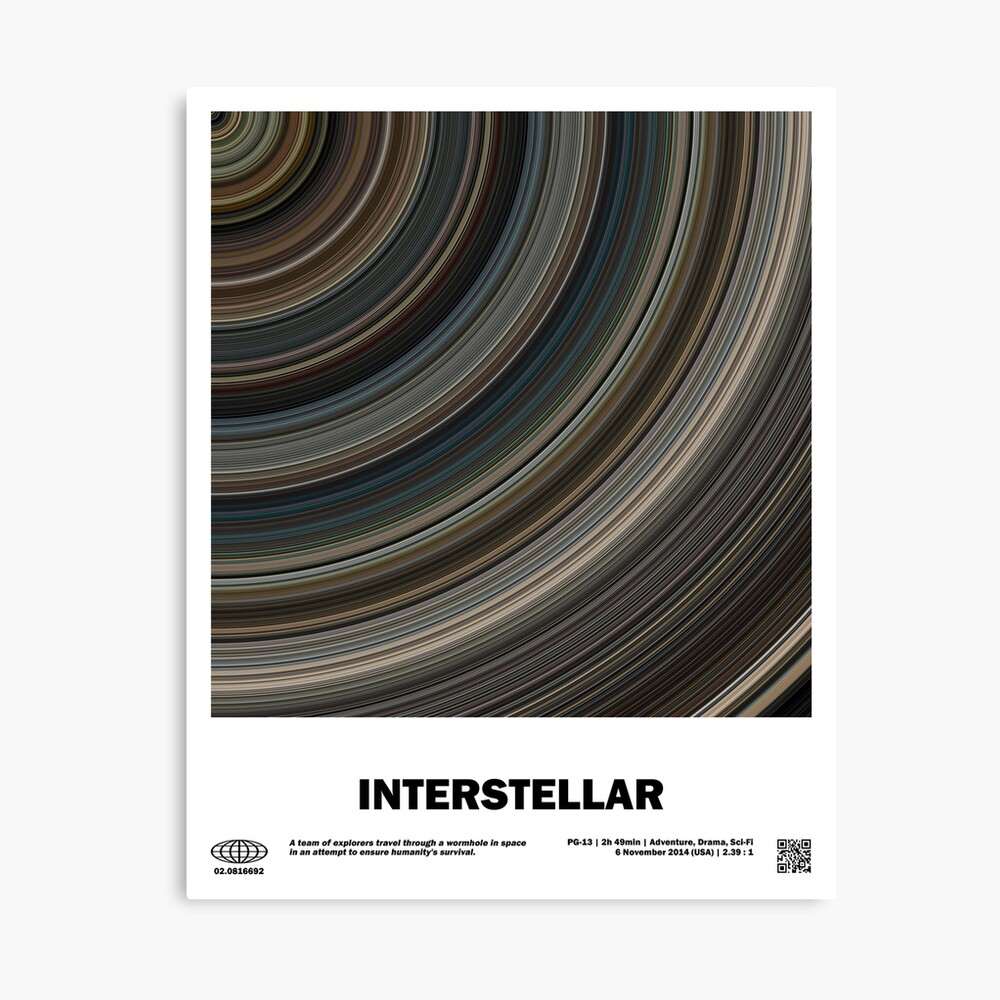The image is a detailed movie poster for "Interstellar," characterized by a retro design evocative of the 1970s. Central to the poster is a top-down view of Saturn's rings, depicted as concentric circles in a myriad of colors including brown, white, blue, turquoise, silver, green, black, and red, creating a visually striking pattern. The bottom of the poster features the film's title, "Interstellar," along with the tagline: "A team of explorers travel through a wormhole in space in an attempt to ensure humanity's survival." Additional details mention that the film is rated PG-13, spans 2 hours and 49 minutes, and falls within the adventure, drama, and sci-fi genres. The release date is noted as November 6, 2014, in the United States. The poster also includes small, hard-to-read lettering and a scannable code, alongside a world-like shape in the corner, further enhancing its interstellar theme.